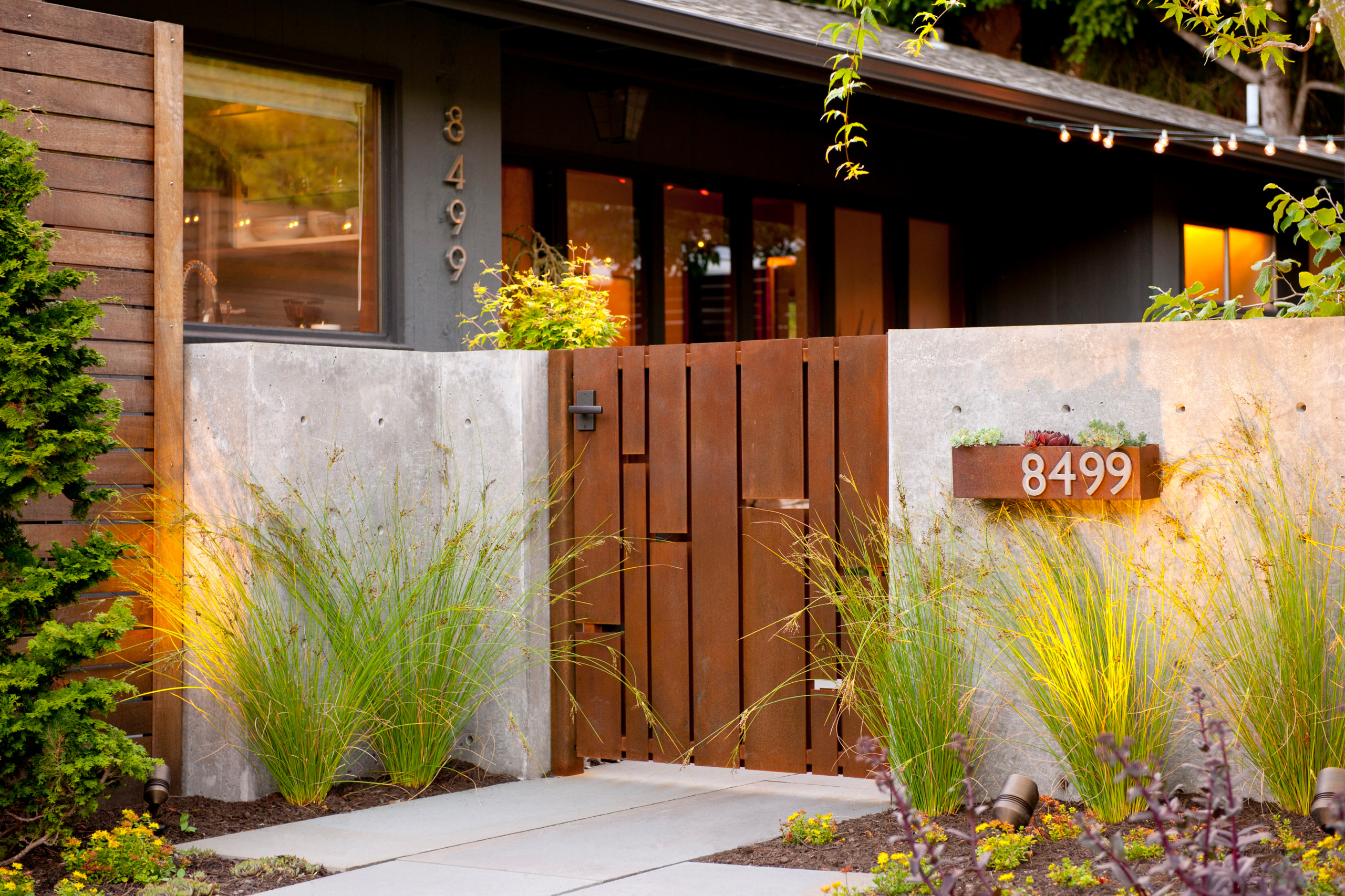This image captures a warm and inviting exterior of a modern home. Central to the scene is a short, waist-level wooden gate with a black handle, firmly set against a sturdy concrete wall. This gate, crafted from a teak-like wood, leads directly into the house, which is painted a sleek gray with brown wood accents, providing a contemporary touch. The address "8499" is prominently displayed twice: once drilled into a wooden number block illuminated by a spotlight on the wall to the immediate right of the gate, and once running vertically next to a picture window and glass entryway on the house itself. Landscaping details include wispy green native lemongrass and vibrant marigolds in a carefully mulched area, enhancing the frontage. To the left, a pretty pine tree adds natural beauty, while café lights strung to the roof amplify the house's inviting ambiance, making it feel exceptionally warm and inviting.